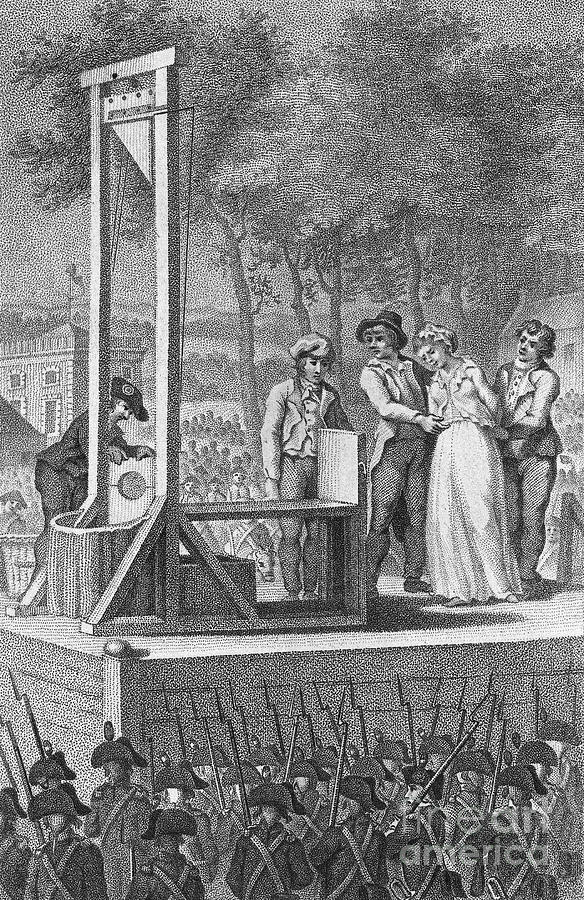This is a detailed black and white drawing depicting a solemn scene from Revolutionary times where a woman is about to be executed by guillotine. In the center of the image, a large elevated platform holds the grim device. The executioner is adjusting the neck portion of the guillotine, preparing for the imminent beheading. The woman, wearing a long dress or gown and a bonnet, stands with her head lowered in sadness and her hands held behind her back by two men, likely guards ensuring she does not escape.

The background features trees with long, slender trunks topped with leaves, while a crowd of spectators gather to witness the execution. This crowd includes a battalion of Revolutionary-era soldiers in military outfits, characterized by their round hats with brims, cross straps, and muskets with bayonets. The soldiers are viewed from the back, standing at attention, their rifles pointed straight to the sky. The entire scene is rendered in shades of charcoal grey and black, intensifying the somber tone of this historic moment.